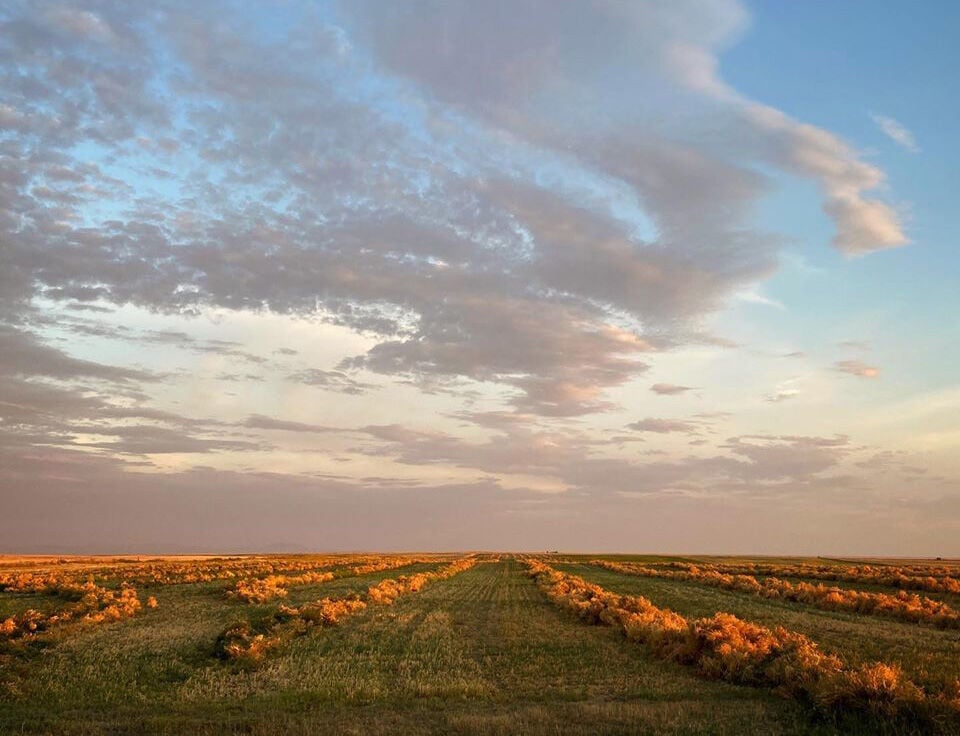This is a color photograph capturing an outdoor scene, likely taken in the early morning or late evening due to the distinctive lighting. The sky is primarily a nice blue color with dark, grayish, and pinkish wispy clouds, which gather more thickly towards the horizon. In the far distance, the faint outline of what might be buildings or a cluster of buildings is just barely discernible. The expansive grassy field in the foreground stretches into the horizon, featuring rows of small, golden-colored bushy plants, spaced far apart with green grass growing between them. These plants stand about 3 feet tall, forming a pattern of furrows. On the left side of the image, there is a hint of shadowy shapes that might be hills or mountains or perhaps just darker clouds. There are also indications of farm equipment at the distant edge of the field, and possibly some tan-colored farm plots to the left, giving the scene a serene, agricultural ambiance.